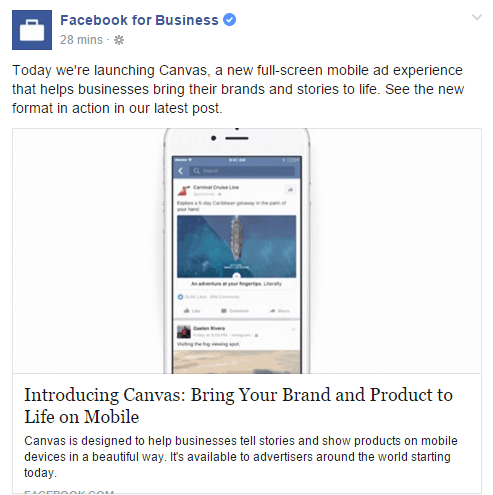A detailed caption for this screenshot might read:

"This screenshot features an article from 'Facebook for Business.' The top section of the image displays the 'Facebook for Business' logo, consisting of a white icon set against a blue background. Next to the logo, the text 'Facebook for Business' is written in bold blue letters on a white background, followed by a white checkmark on a blue backdrop. Below this header, the timestamp '28 minutes' indicates the recency of the post. The article headline announces, 'Today we're launching Canvas,' positioned above a brief description of Canvas, described as a tool for creating engaging ads. Following the introductory text is a photograph of a smartphone, exemplifying the mobile-focused nature of Canvas. The body of the article elaborates with the title, 'Introducing Canvas: Bring your brand and product to life on mobile,' before continuing into a more detailed exposition about the features and benefits of the Canvas tool."